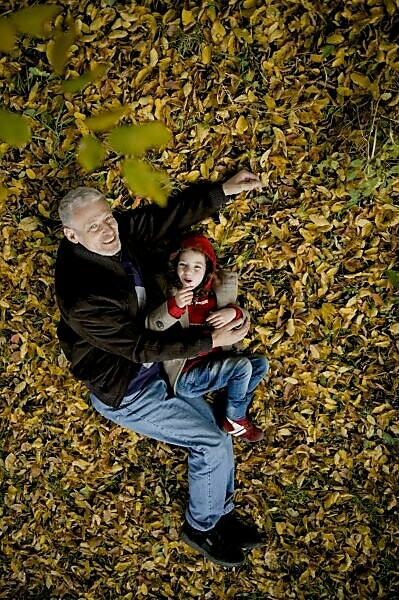In an enchanting autumn scene, captured from high above, a photograph showcases a heartwarming moment between a man, possibly a dad or grandpa, and a young boy around four or five years old. They are lying on a blanket of yellow leaves, with no grass visible beneath. The man, with gray hair, is dressed in a black coat, blue jeans, and black tennis shoes. He holds the boy close with one arm while the boy, wearing a tan coat over a red hoodie, blue jeans, and red shoes with white decorations, nestles beside him. The boy is captured mid-bite, with something in his hand, which adds a natural and candid charm to the scene. Both are joyfully looking up toward the camera, their laughter radiating happiness. The leaves around them, recently fallen and unspoiled, suggest the peak of the autumn season. The perspective, possibly from a drone or a high vantage point like a tree, adds a unique and captivating angle to this tender moment. Blurred green leaves and branches in the foreground hint at the environment beyond, framing this idyllic and intimate snapshot of joy and togetherness amidst nature's autumnal display.